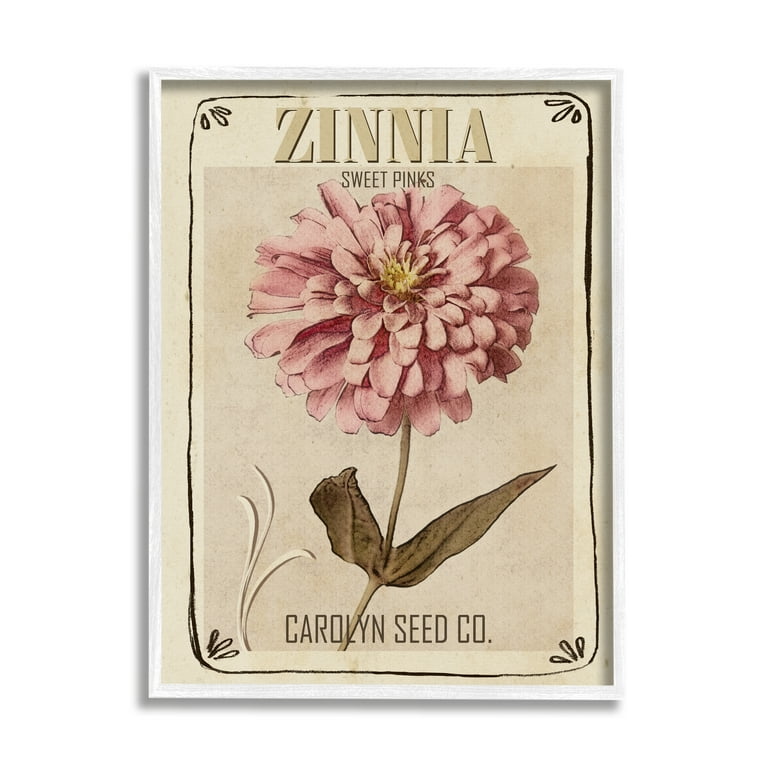This image features a framed print designed to resemble an old-fashioned seed packet. The frame is a thin, white wooden rectangle, positioned vertically and enclosing the artwork. The print has an aged, beige background, evoking a vintage aesthetic. 

At the top of the design, "Zinnia" is prominently displayed in bold beige lettering with a black outline. Below this title, there is a detailed illustration of a zinnia flower. The flower has numerous small, oval-shaped, pink petals radiating outwards from a yellow center. Attached to the flower is a green stem with two green leaves.

Further down, text in a dark color reads "Sweet Pinks". At the very bottom of the print, "Carolyn Seed Co." is inscribed, also in a dark color. The entire illustration is enclosed within a hand-drawn, rectangular border with slightly curved corners, featuring small embellishments or oval-shaped leaves at each of the corners. This elaborate design contributes to the nostalgic feel of the overall presentation, reminiscent of seed packets from the 40s or 50s.